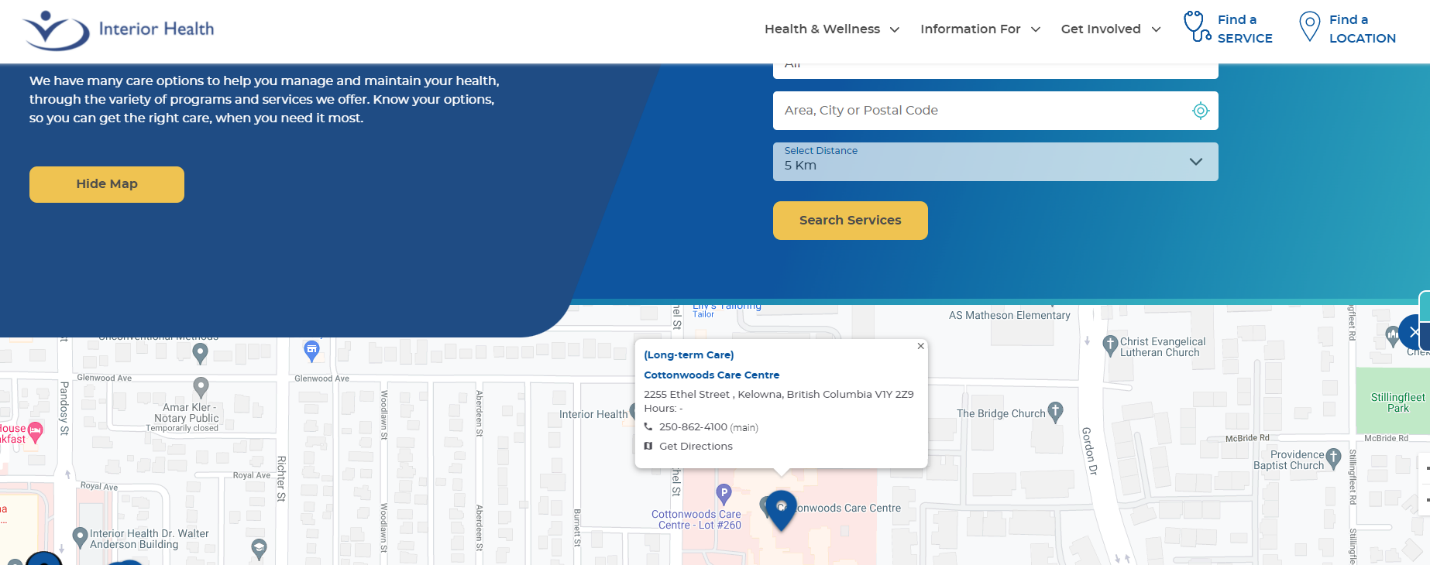Screenshot of the Interior Health Website:

The screenshot showcases the homepage of the Interior Health website, which is dedicated to health and wellness services. In the top left corner, the title "Interior Health" is prominently displayed. Across the top navigation bar, there are several drop-down menus labeled "Health and Wellness," "Information For," and "Get Involved." Additionally, options to "Find a Service" and "Find a Location" are situated on the far right of the navigation bar.

Beneath the navigation bar, on the left side of the screen, there is a message stating: "We have many care options to help you manage and maintain your health through the variety of programs and services we offer. Know your options so you can get the right care when you need it most." Below this message, there is a yellow "Hide Map" button.

The central section of the screen features a large blue rectangle containing several fields for users to input information. These fields include prompts for city, state, postal code, and a distance parameter set to 5 kilometers. There is also a "Search Services" button, which acts as a go button for the search functionality.

Below the blue rectangle, a map is displayed, pinpointing the location of "Long-term Care Cottonwoods Care Center," located at 225 Ethel Street, Kelowna, British Columbia, Canada.